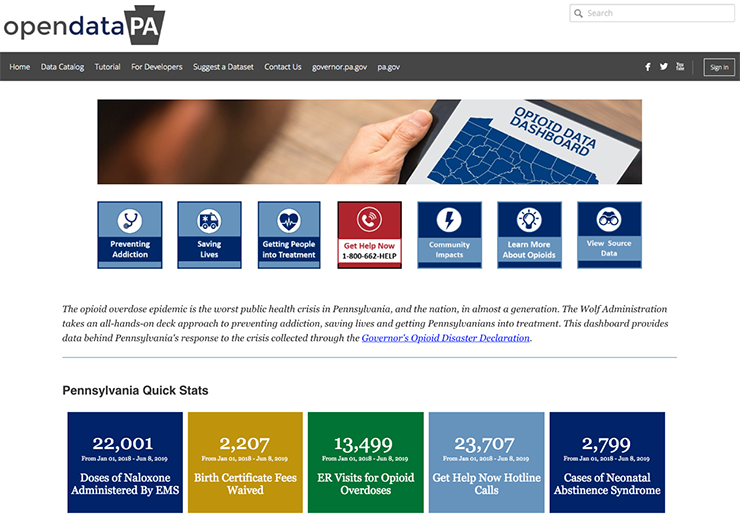Here's a detailed and cleaned-up caption for the described image:

---

A detailed screenshot of the Open Data PA webpage, featuring a black navigation bar with options including Home, Data Catalog, Tutorial for Developers, Suggest a Data Set, Contact Us, Governor, Pennsylvania, GOV, and PA.gov. The top-right corner contains icons for Facebook and Twitter, along with a sign-in box. Just beneath the menu bar is a panoramic image displaying a hand holding a notebook labeled "Opioid Data Dashboard." Below the image, blue rectangles outline key initiatives: "Preventing Addiction," "Saving Lives," "Getting People Into Treatment." A red box prominently reads "Get Help Now." Additional blue boxes offer more options such as "Community Impact," "Learn More About Opioids," and "View Source Data."

A paragraph beneath these boxes highlights the severity of the opioid overdose epidemic in Pennsylvania and the nationwide response, emphasizing the Wolf Administration's comprehensive strategy to address this crisis. It explains that the data on the dashboard is collected through the Governor's Opioid Disaster Declaration.

At the bottom of the page, four different color-coded rectangles display critical statistics: 

- In gold, "2,207 birth certificate fees waived."
- In green, "13,499 ER visits for opioid overdoses."
- In light blue, "23,707 Get Help Now hotline calls."
- In dark blue, "2,799 cases of Neonatal Abstinence Syndrome."

Also noted are the "22,001 doses of Naloxone administered by EMS."